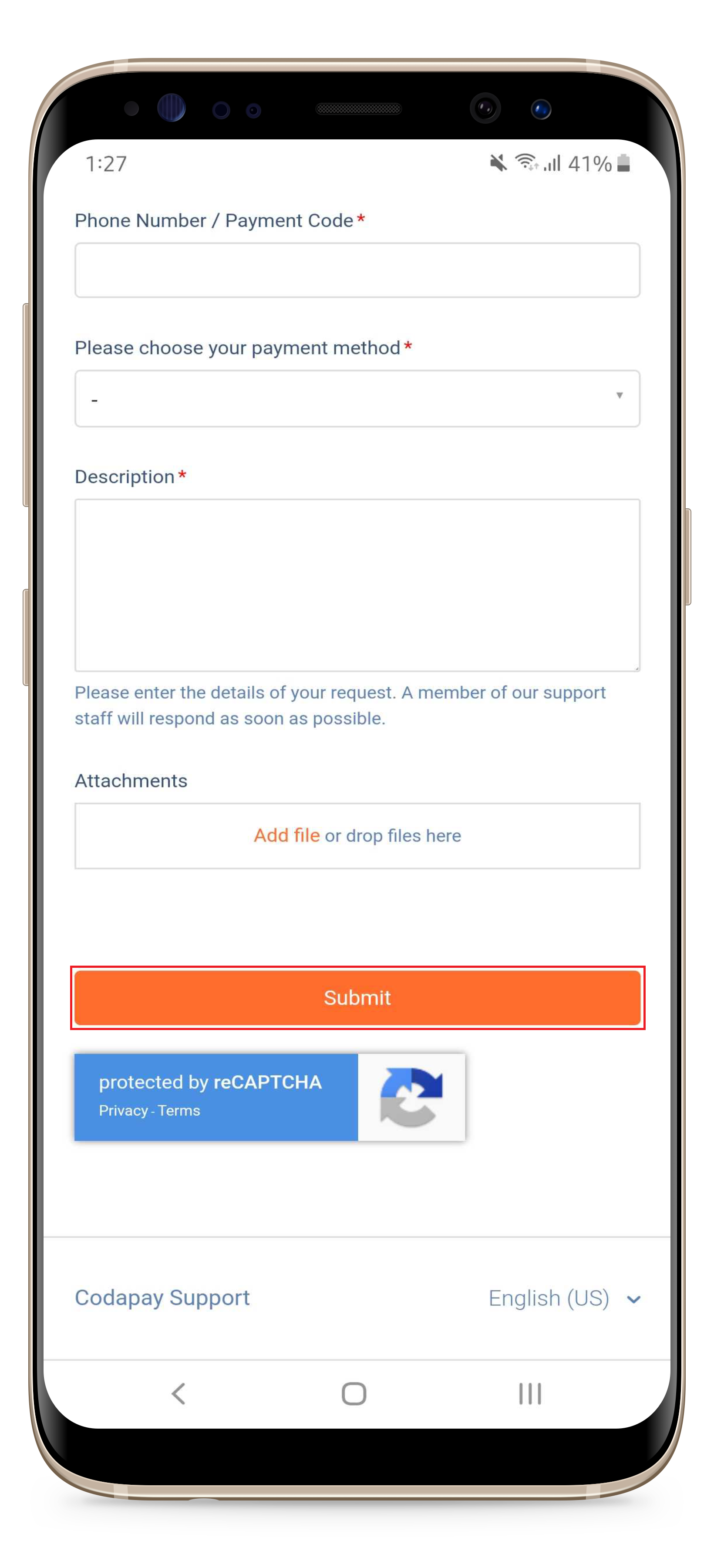The image shows a phone screen with various UI elements:

1. At the top of the screen, there's a black bar containing grey and blue buttons.
2. In the white area at the top, the number "127" is displayed, accompanied by a symbol that is not clearly identifiable, followed by a WiFi symbol composed of four progressively longer lines.
3. The battery level indicator next to these symbols shows 41%, indicated by a partially filled grey battery icon.
4. Below this, a blue text reads: "**Phone Number / Payment Code**," marked with a red asterisk, with a text box underneath for input.
5. Further down, the text reads: "**Please choose your payment method**," also marked with a red asterisk, followed by another text box.
6. After that, the word "**Description**" appears with another red asterisk, followed by a larger input box.
7. Below the description box, there's an instruction: "**Please enter the details of your request. A member of our support staff will respond as soon as possible**."
8. There is a section titled "**Attachments**," which includes a prompt to "**Add file**" in red or to "**drop files here**" written in blue.
9. At the bottom, there is an orange submit button with a white outline and inner text reading "**Submit**."
10. Beneath the submit button, there is a note stating: "**Protected by 3 Kappa Chia Privacy Terms**," with an adjacent white box containing a circular arrow icon made up of three arrows.
11. A grey line divides this section from the bottom, where it states: "**CODA Pay Support**."
12. On the right side of the bottom part, there is a language selection option showing "**English (US)**" with a downward arrow, and below it, an icon with a right-pointing arrow, a square, and three lines.